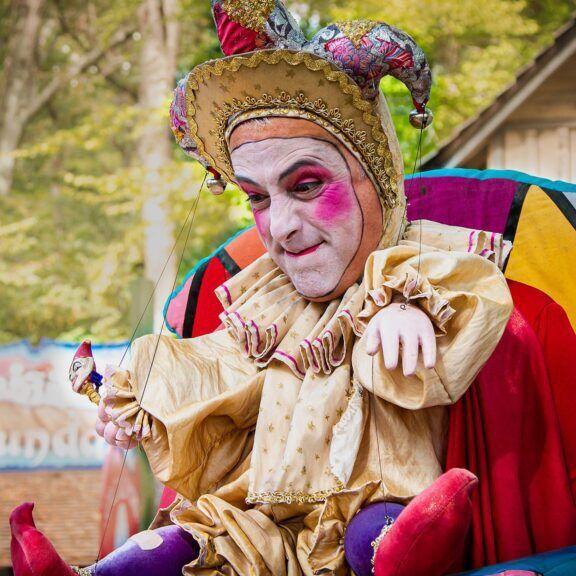The image depicts a person, presumably a man, dressed as a French court jester in a vibrant and theatrical costume. His face is painted white with bright red lipstick, pink cheeks, and pink eyeshadow, resembling a marionette puppet. He wears a jester's cap that has three points with bells at the ends. His attire includes a poofy, cream-colored, frilled shirt, purple pants, and red-tipped shoes. Strings extend from his jester's cap to the arms and legs of the costume, giving the impression that he is part of the puppet. In his hand, he holds a jester's wand. His head appears disproportionately large comparing to the puppet-like body, suggesting he is behind it to give an illusion of a toy. The scene is likely outdoors with a colorful blanket in the background, amidst trees and what appears to be the roof of a wooden house, indicating it could be part of a parade or a play, possibly connected to New Orleans' Mardi Gras festivities.